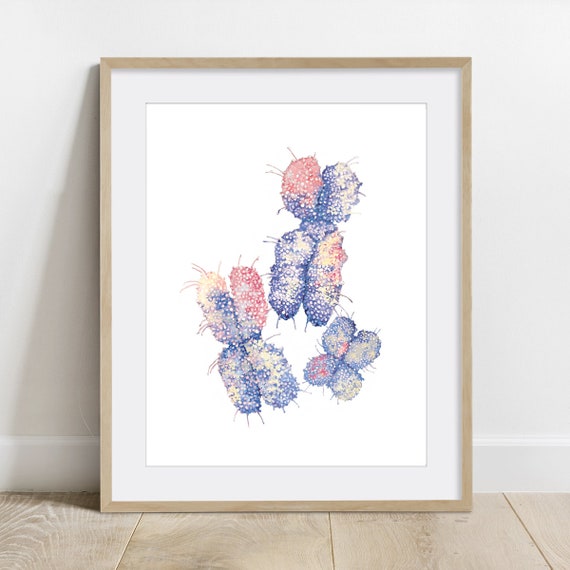In this photograph, a painting rests on a light brown wooden floor, leaning against a stark white wall. The painting, encased in a matching light brown wooden frame, features three vibrant, multicolored, chromosome-shaped figures that could also be interpreted as abstract butterflies or bugs, rendered in shades of blue, red, orange, and a hint of yellow. These figures are set against a clean, white background, creating a striking contrast. The composition gives the impression of these whimsical, feeler-adorned shapes flying or floating in various directions across the canvas. The painting's placement casts a shadow to the left, and a white trim runs along the base of the wall where it meets the floor.